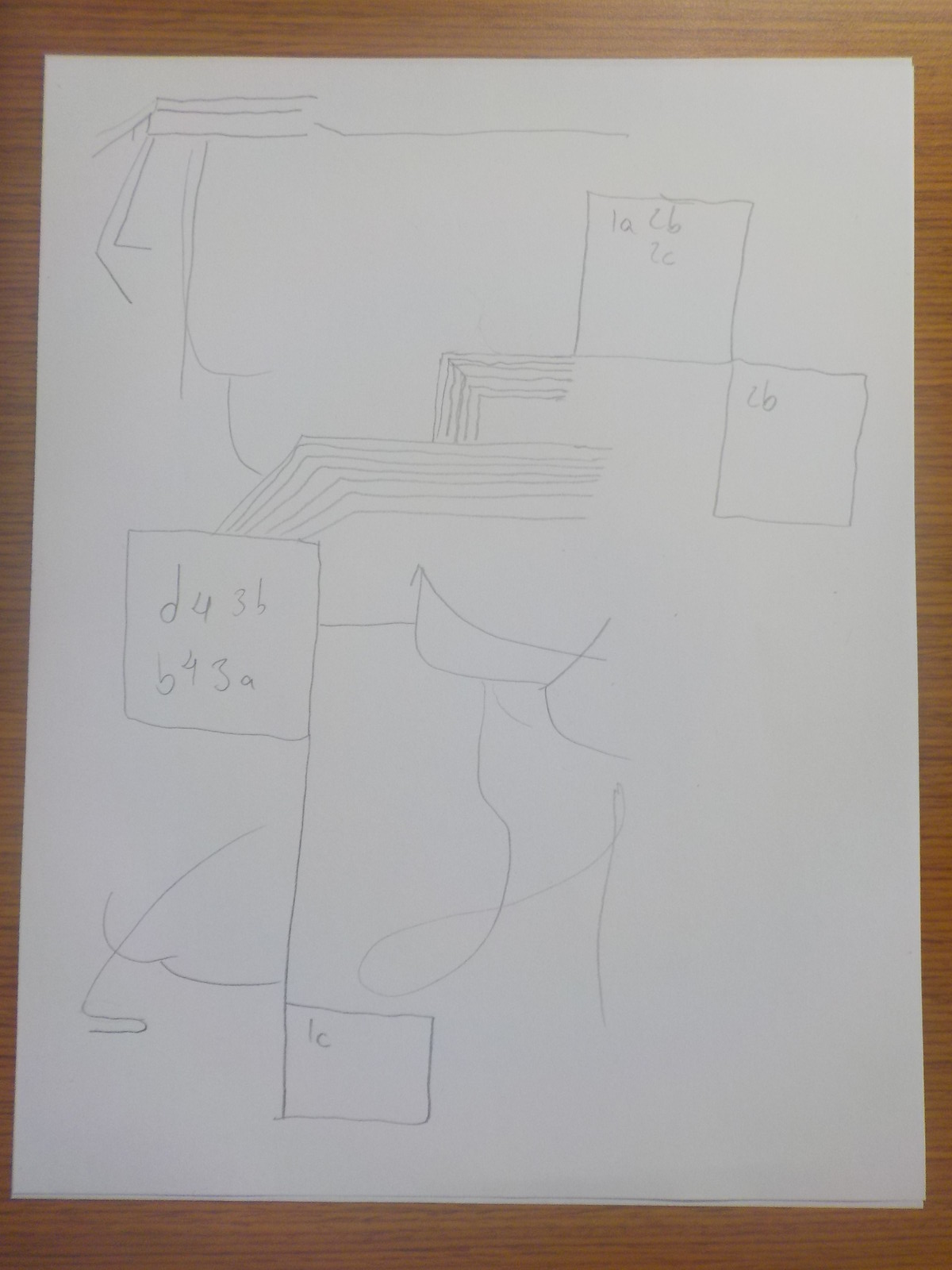This image showcases a white sheet of standard computer paper positioned against a smooth, medium-brown wooden surface, displaying prominent wood grain patterns. The setting appears to be indoors with natural lighting, as there is no indication of artificial lights being used.

The paper features a rough sketch, likely hand-drawn. In the top left corner, three parallel lines are visible. These lines attach to two parallel lines curving downward into L shapes. These L-shaped lines connect to another series of L-shaped lines, ultimately linking to a box. Inside this box, inscriptions read "1A," "2B," and "2C" in the bottom right corner, while the top left specifies "2B."

From this box, a complex network of L-shaped lines extends to another box containing the numbers "2D," "4," "3B," "B," "4," and "3A." This lower box branches off into a boat-like shape to the right, with a connecting line extending downward to another smaller box labeled "1C." Additionally, there are some unclear, squiggly lines emerging from the bottom of this smaller box, which may either be part of the illustration or extraneous marks made by the artist.

In summary, the image appears to be a conceptual diagram or sketch with a series of interconnecting boxes and lines labeled with numbers and letters, all set against a finely textured wooden background.